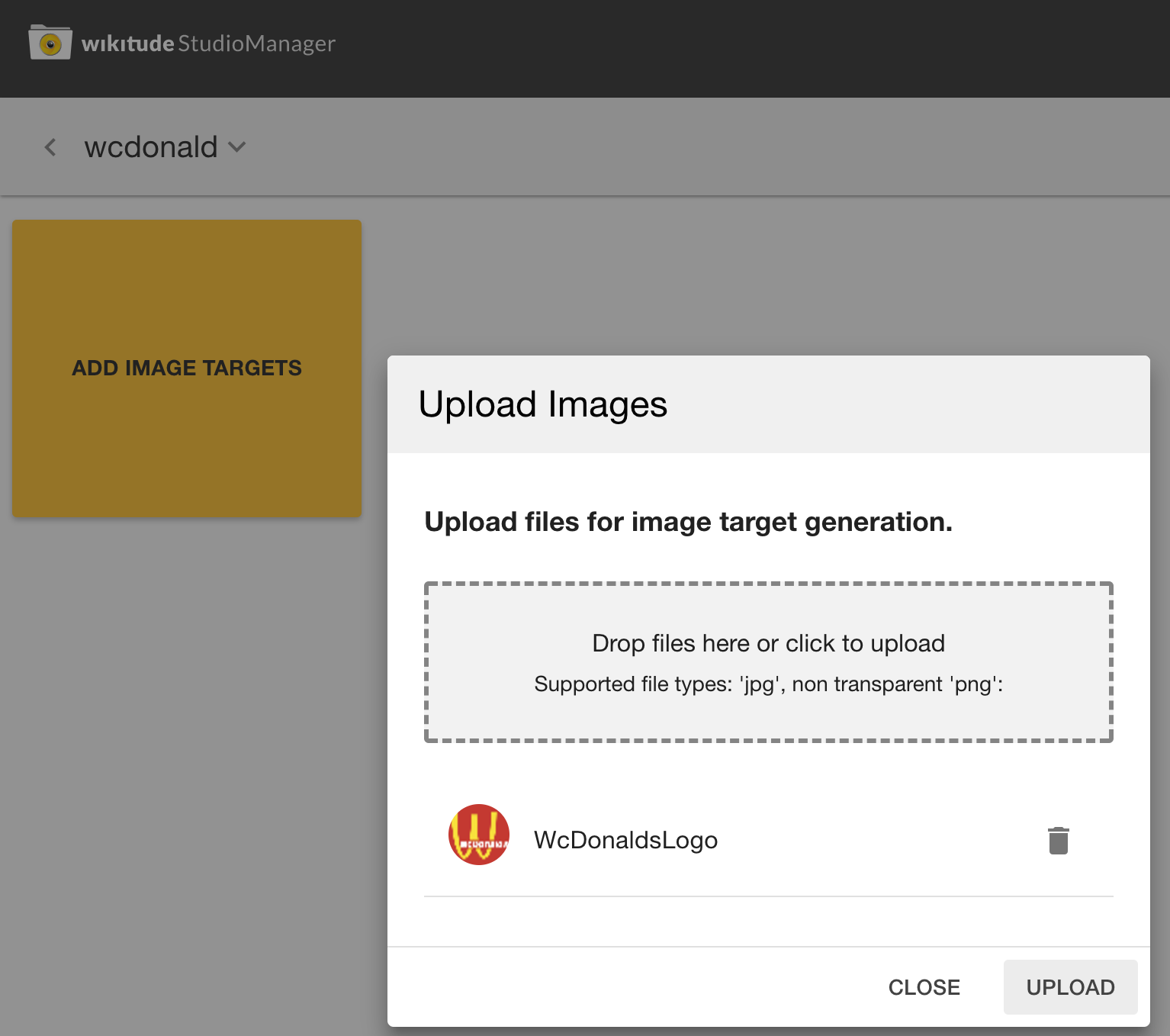The image depicts a website with its main interface grayed out due to the presence of a pop-up window. The primary section of the website appears sparse, with minimal visible content. In the top left corner, there's a back arrow, possibly allowing users to return to a previous page. Next to the arrow, the text "W.C. Donald" is displayed, accompanied by a downward arrow suggesting a drop-down menu option.

Directly beneath this is a small, rectangular, yellow-orange box, though it too is slightly grayed out. Inside this box, in black lettering, the text reads "Add Image Targets." This appears to be the extent of the content visible on the original homepage.

The pop-up window itself has a gray border at the top, highlighting its header. The header text in black reads "Upload Images," followed by the bold text "Upload Files for Image Target Generation." Below this, there is a prominent gray box outlined with dotted lines, indicating a drop zone for files. The text within this box instructs users to "Drop Files Here or Click to Upload" and specifies the supported file types: "JPG, Non-Transparent, PNG."

Below the upload box, an image file appears to have been uploaded. The image is the McDonald's logo, but it is displayed upside down, making the 'M' appear as a 'W.' The accompanying text reads "Wc W. Arnold's logo," with unusual capitalization. At the very end of the row, there is a small trash can icon, possibly for deleting the uploaded file, and buttons labeled "Close" and "Upload" are visible, offering options to finalize the action.